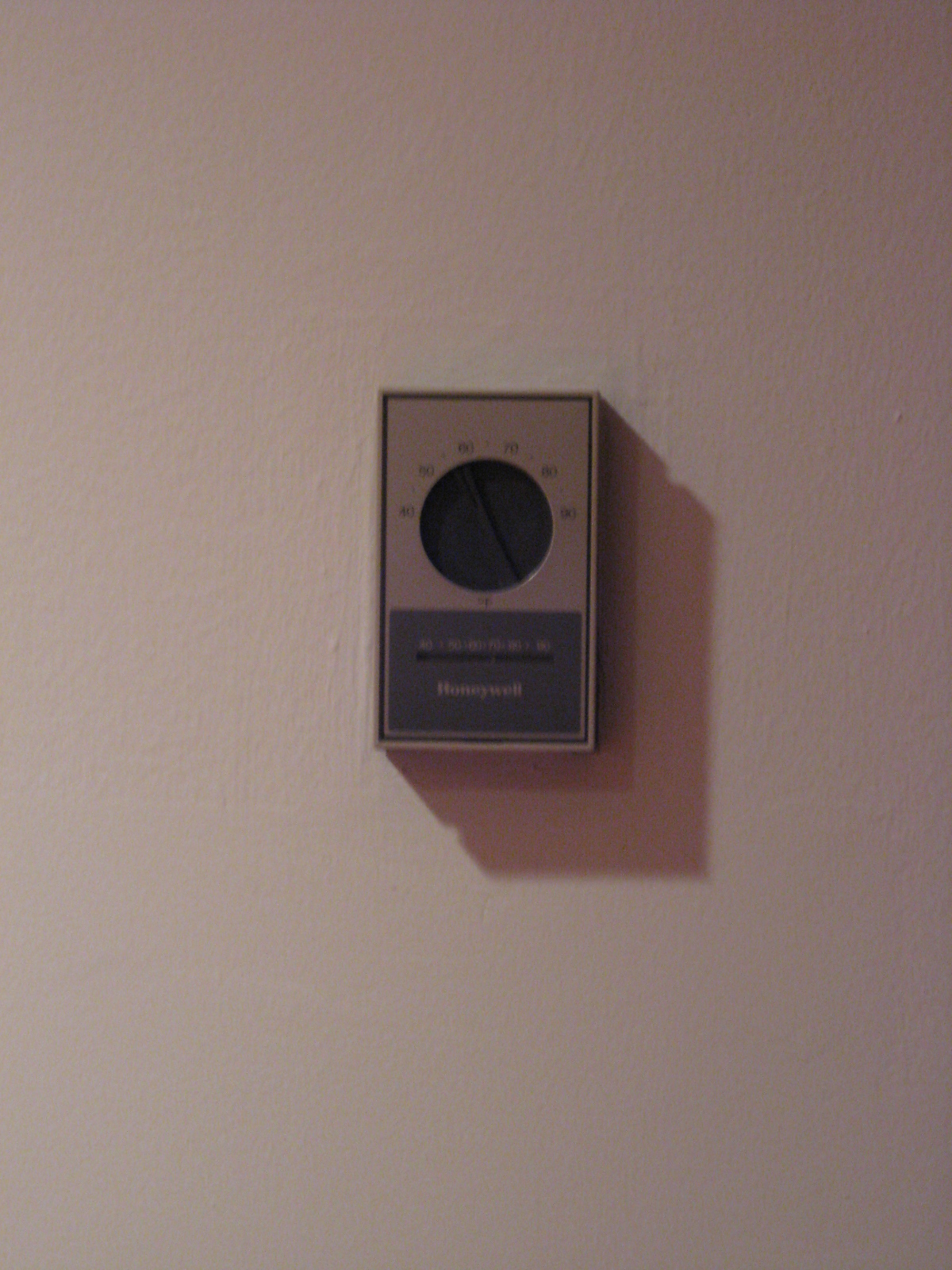In this dimly lit photo, we see an old-fashioned thermostat mounted on a beige-tan wall within what appears to be an older home. The image has a warm, low-light ambience, which casts a subtle shadow of the thermostat onto the wall. The thermostat itself is rectangular, blending in with the wall due to its similar beige-brown metallic color. At the center of the thermostat is a circular dial with black markings, displaying temperature settings ranging from 40 to 90 degrees Fahrenheit. Despite the blur, one can make out the numbers positioned around the dial. Below the dial is a gray rectangle bearing the "Honeywell" logo, although additional text below the brand name remains unreadable due to the blurriness of the image. The simplicity of the scene, combined with the dim lighting, evokes a nostalgic feeling, hinting at the thermostat’s importance within a quieter, possibly vintage household setting.